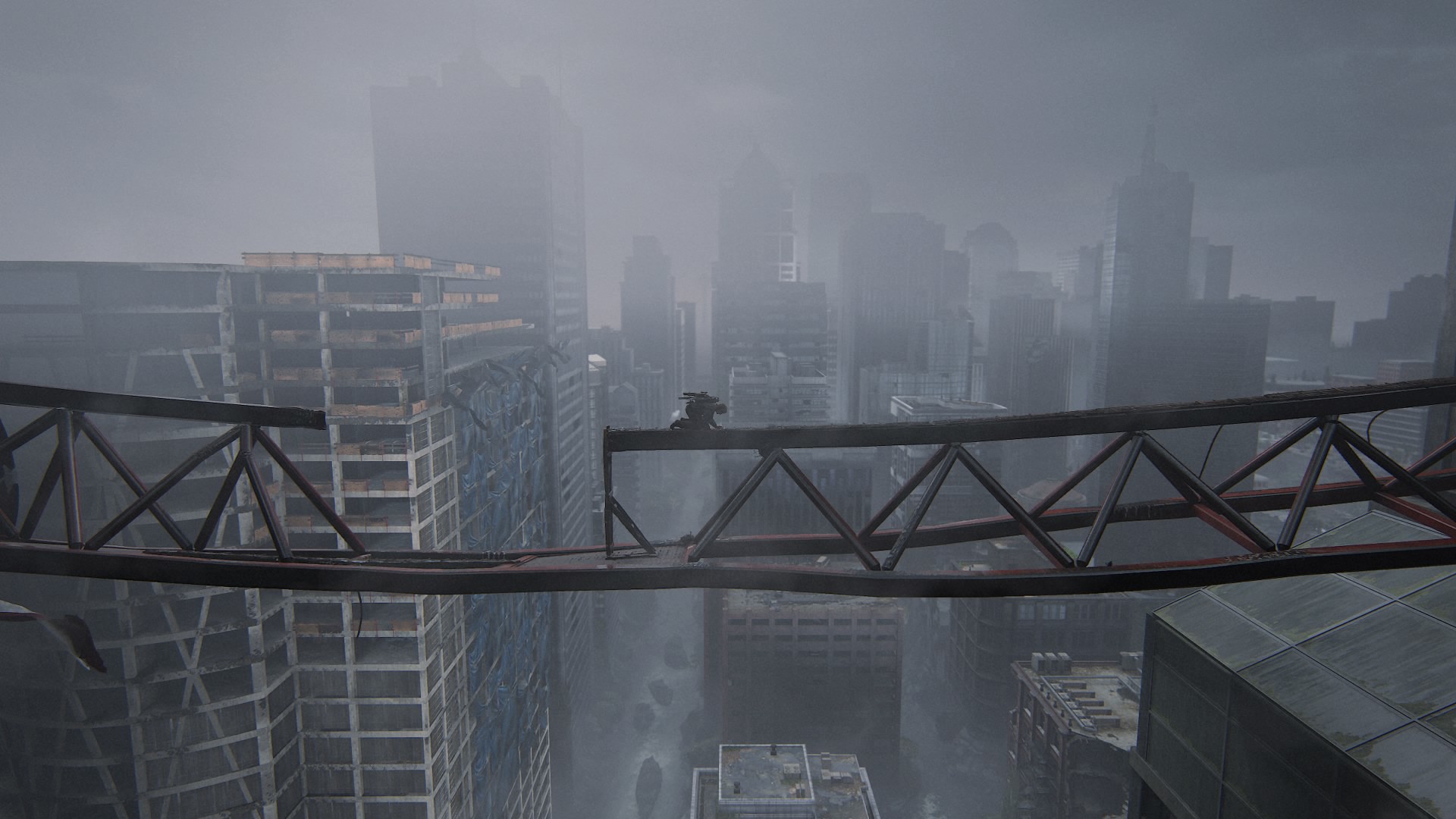The image depicts a fog-drenched, post-apocalyptic cityscape, characterized by damaged and deteriorating structures. A metal beam, evidently broken on the left side, hangs precariously across the scene, with a small black silhouette—possibly a person—perched on top of it. To the left, a tall, worn building stands, its dilapidated state echoed by other crumbling skyscrapers visible in the background. The overcast sky and thick mist obscure the city's horizon, intensifying its somber and desolate atmosphere. Vehicles scattered along the road hint at the city's once bustling nature, now reduced to a haunting remnant of civilization, reminiscent of scenes from "The Last of Us Part II."